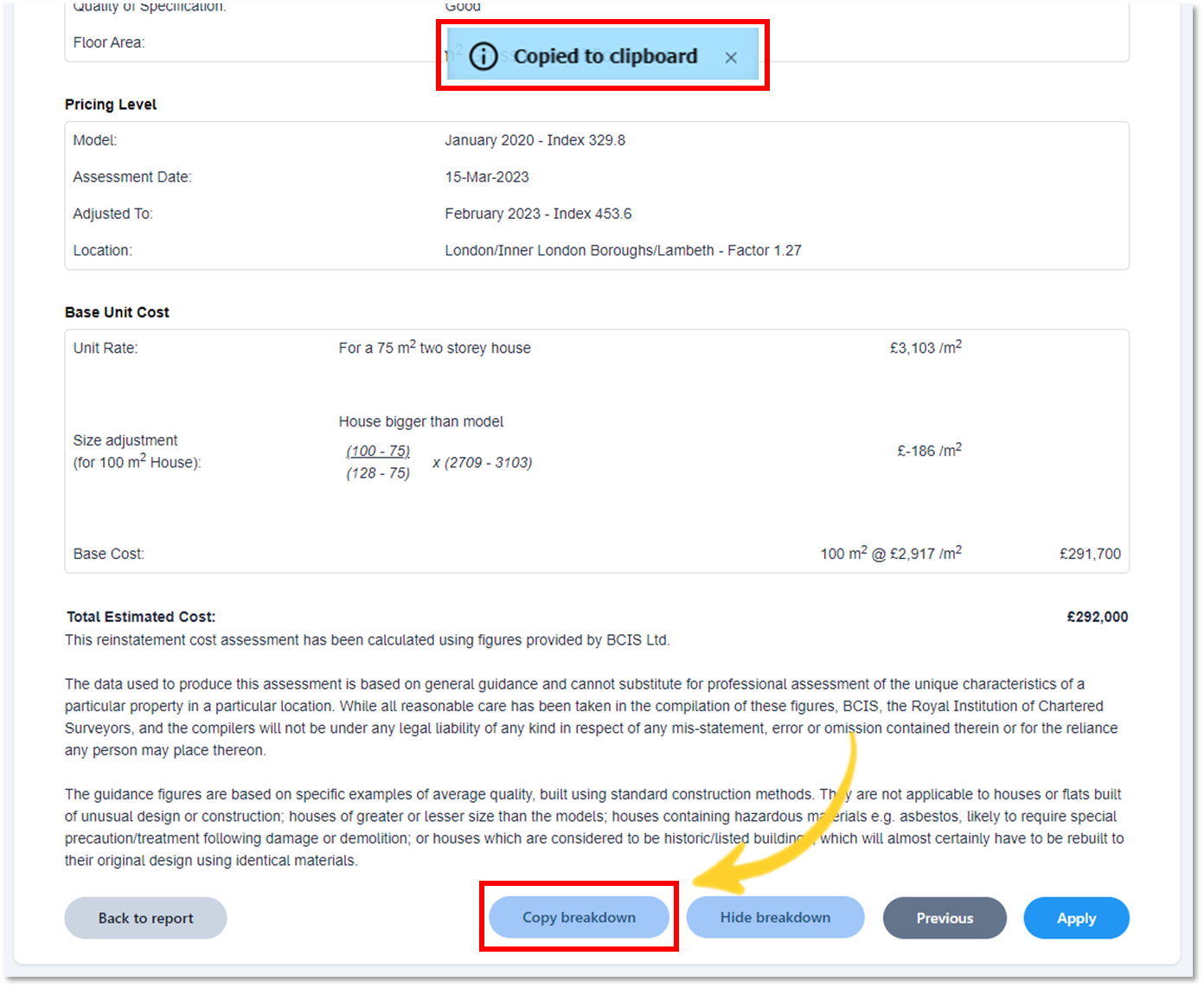**Detailed Invoice Breakdown Screenshot with Highlighted Pop-up**

This image is a partial screenshot of a price breakdown document, showcasing the bottom portion of the page. Dominating the top center of the frame is a blue pop-up notification that reads "Copied to clipboard," accentuated by a prominent red rectangle around it for emphasis. The document itself is spread over a crisp white background, segmented into multiple sections each bordered by thin gray lines for clarity.

**Section 1: Pricing Level**
- **Pricing Level:** Includes four distinct lines of information:
  1. **Model:** January 20 to index 329.8.
  2. **Assessment Date:** 15 March 2023.
  3. **Adjustment to February 2023 Index:** 453.6.
  4. **Location:** London/Interlondonborough/Lambeth-factor 1.27.

**Section 2: Base Unit Cost**
- **Base Unit Cost:** Comprising several sub-items:
  1. **Adjustment Rate for a 75 Square Meter Two-Story House:** £3,103 per meter squared.
  2. **Size Adjustment for 100 Square Meter House Calculation:** 
    - Formula: \( \frac{100-75}{128-75} \times (279-3109) \).
    - Result: \( -£186 \) per square meter.
  3. **Base Cost Calculation for 100 Square Meters:** 
    - Rate: £2,917 per square meter.
    - Total Cost: £291,700.

**Final Statement: Total Estimated Cost**
- The concluding line of the document states: "This reinstatement cost assessment has been calculated using figures provided by BCIS limited."
- **Total Estimated Cost:** Boldly highlighted to the right: £292,000.

This descriptive breakdown ensures each section and calculation is detailed for a clear and comprehensive understanding of the document's contents.